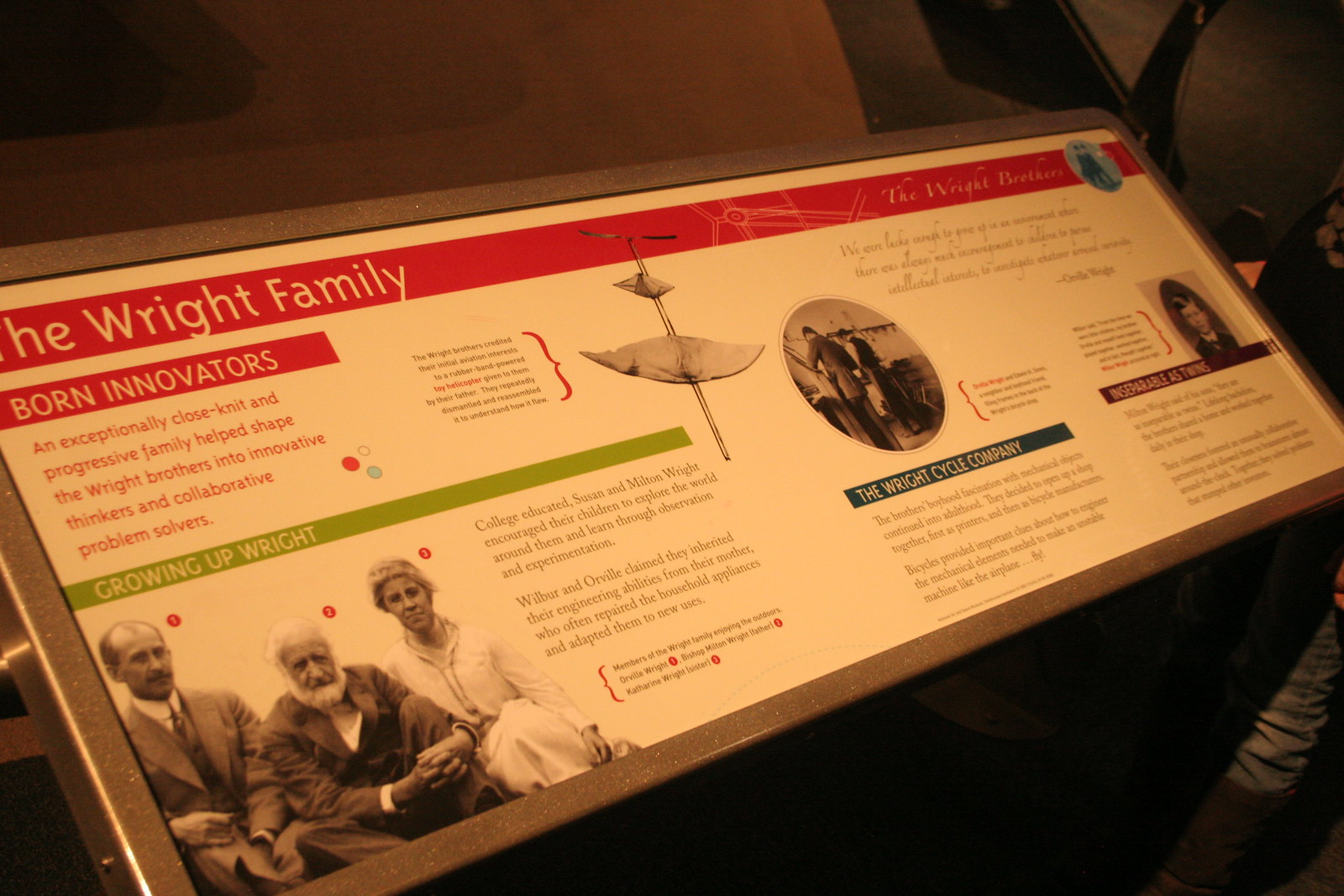This image depicts a detailed museum plaque dedicated to the Wright family, showcasing their significant contributions to aviation history. The plaque is wide and rectangular, mounted within a thick gray metal frame, and positioned at an angle with the left side closer than the right. It has an off-white background with vibrant headings in red, green, blue, and purple, providing a colorful contrast against the monochromatic photographs.

At the top, a long red rectangle with white font proudly reads "The Wright Family," highlighting their legacy. Directly below, a smaller red rectangle states "Born Innovators," emphasizing their creative and forward-thinking nature. Further down, a green line reads "Growing Up Right," indicating a section dedicated to the Wright family’s upbringing.

The plaque features several black-and-white photographs, including three people seated, with one man sporting a long gray beard, and a woman in an old-fashioned white dress. In the center, a larger image shows two individuals working in a workshop, their backs turned to the viewer, symbolizing their collaborative spirit. To the right of this central image is a portrait of a young boy, suggesting an early stage of the Wright family’s journey.

Additionally, there's an area depicting an old-timey flying device, further illustrating the Wright brothers' groundbreaking achievements in aviation. The entire exhibit, with its mix of historical photos, bold text, and vivid colors, serves as a tribute to the Wright family's innovative legacy and their pivotal role in shaping modern flight.